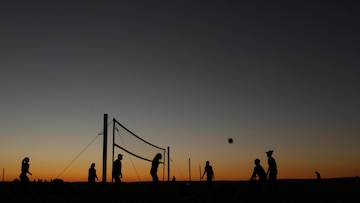This image captures a dynamic scene of silhouetted figures engaged in a spirited game of volleyball on the beach during an evocative sunset. Taken from a low vantage point, the shot immerses the viewer in a moment where the sky transitions from a dark, starless blue to a deep, dark gray as night approaches. The horizon is tinged with a dark, orangish-yellow glow, casting just enough light to highlight the black silhouettes of seven people energetically playing volleyball—four on one side of the net and three on the other. Above them, the volleyball is suspended mid-air, tense with the anticipation of a forthcoming hit. The net, clearly discernible with its attached poles and supporting strings tied to stakes, stands as a stark silhouette against the fading light. In the distance, another volleyball net is faintly visible, marked by two barely perceptible poles, accompanied by two stationary figures. The ground beneath the players is a solid black, emphasizing the twilight setting and the striking contrast created by the diminishing daylight.